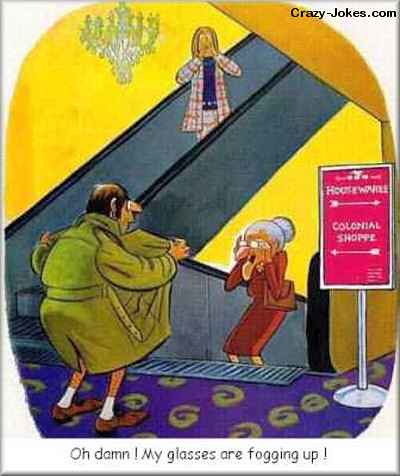The image is a portrait-oriented, vibrant, color illustration depicting a humorous and satirical scene reminiscent of a one-panel comic. At the center, an elderly woman with her white hair pinned up in a bun ascends an escalator. She is dressed in a red dress and wears glasses, which are emphasized by the caption at the bottom of the image that reads, "Oh Damn! My glasses are fogging up!" 

To the left, at the top of the escalator, a man in a green trench coat is flashing her, provocatively opening his coat. The woman has a shocked expression on her face as she looks directly at him. Above her, another escalator hosts a second woman who is covering her eyes with her hands, likely in disgust or to avoid seeing the indecent act below. The background of the image is primarily yellow, adding to its cartoonish style, with a red directional sign visible on the right side of the escalator.

In the top right corner, the black text "crazyjokes.com" is placed, and a subtle white border frames the entire illustration. The overall style and elements suggest that this image is designed to be a light-hearted, shareable meme for social media. Various colors such as white, black, purple, green, brown, pink, and silver are prominently featured throughout the image, adding to the detailed and lively appearance of the artwork.